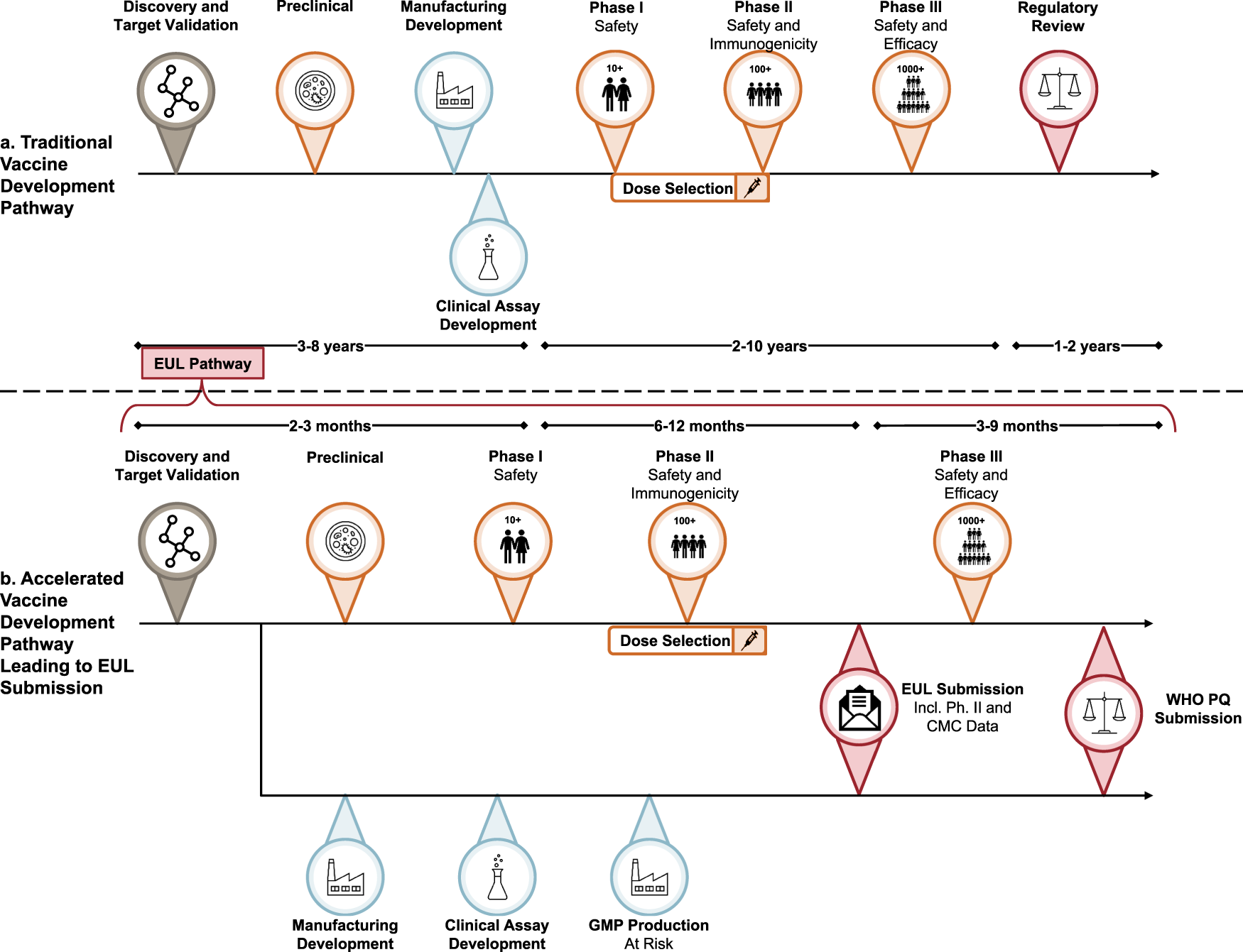The image is a detailed infographic with a white background, illustrating two pathways for vaccine development: the traditional vaccine development pathway and the accelerated vaccine development pathway leading to EUL submission. Across the top, the title "Traditional Vaccine Development Pathway" is displayed in black, followed by a left-to-right timeline that includes the stages: discovery and target validation, preclinical, manufacturing development, phase one safety, phase two safety and immunogenicity, phase three safety and efficacy, and regulatory review.

Beneath this traditional pathway, the infographic features another timeline labeled "Accelerated Vaccine Development Pathway Leading to EUL Submission," marked by a prominent red rectangle indicating "EUL Pathway." This pathway is more complex, incorporating additional details and steps. It begins similarly with discovery and target validation, preclinical, phase one safety, phase two safety and immunogenicity, phase three safety and efficacy. It then includes unique stages such as dose selection, manufacturing development, clinical assay development, and GMP production at risk before reaching EUL submission, which encompasses phase two and CMC (Chemistry, Manufacturing, and Controls) data, followed by WHO PQ submission.

The chart timestamps various stages, indicating periods ranging from three months to over ten years. The infographic’s clean design uses multiple lines and circles to connect these stages, making the complex process visually comprehensible.